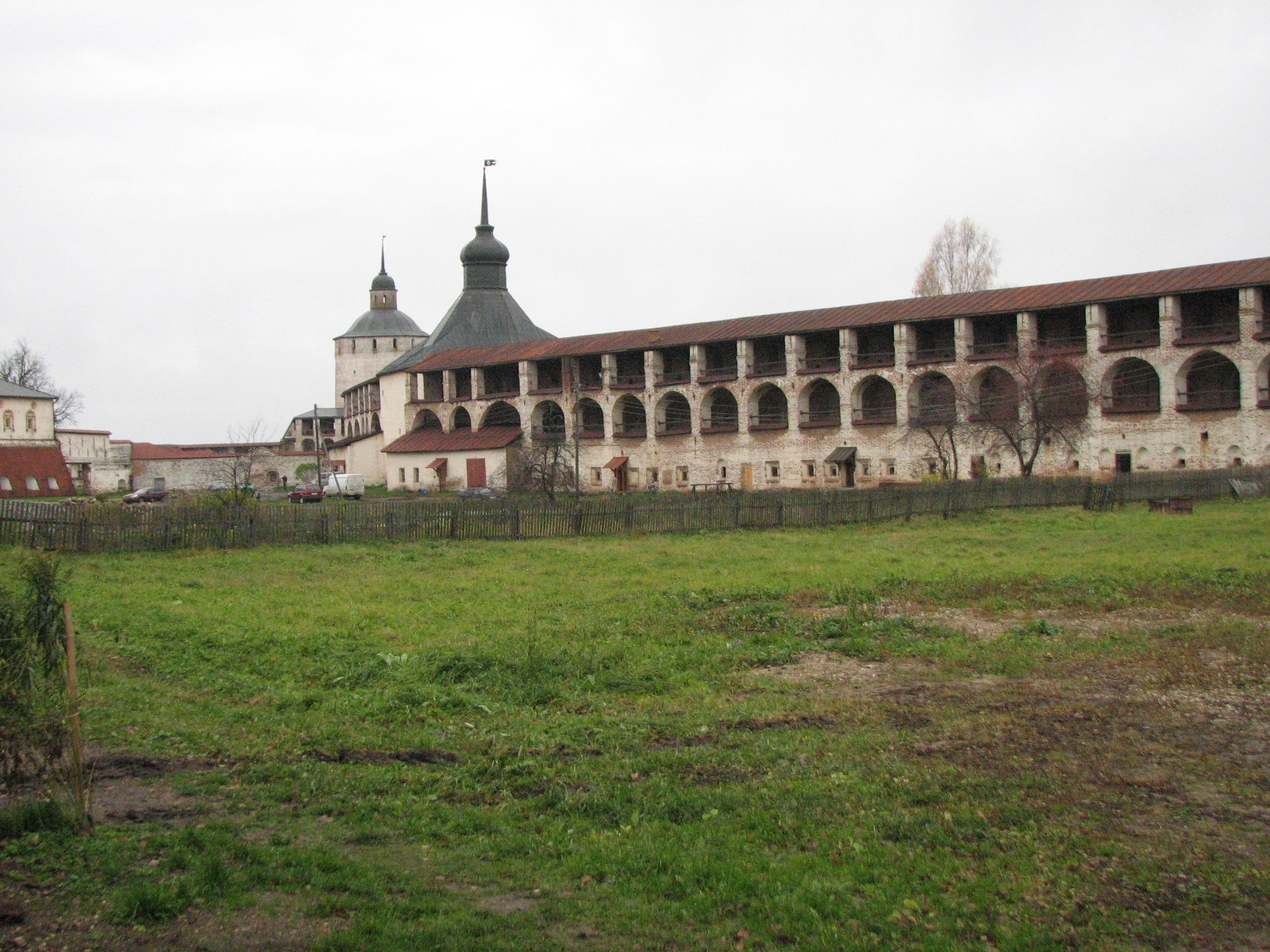The image captures a sprawling Spanish-style building complex, likely abandoned, under an overcast sky. The primary structure is notably long and stretches across the frame. Its architecture features a ground floor topped by a series of arches, with pillars supporting the ceiling above. The left end of the building is marked by a conical spire with a flag flying at its peak. In the vicinity, a similar round building with a matching spire rises up, flanked by a row of low, attached structures. The entire complex is enclosed by a wooden fence, and a couple of cars are faintly visible in the courtyard. The foreground consists of unkempt grass and patches of dirt, adding to the sense of abandonment. The predominant colors are brown, green, and gray, reinforcing the subdued, historic ambiance of the setting.